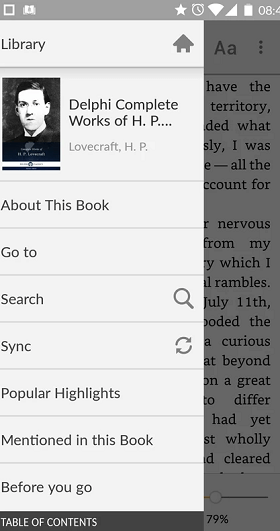This image is a vertically oriented rectangular snapshot, likely taken from a smartphone. The image has a light gray border at the top. On the right side, there is a white box with a gray center, followed by an unidentifiable icon. Moving to the right towards the center, there is a row of icons, including a star, an alarm clock, a full Wi-Fi signal indicator, a full cell phone service signal indicator, and a nearly full battery charge icon. The visible part of the time reads "08:4."

Towards the bottom of the image, there appears to be a pop-up window overlaying another window. This pop-up window is cut off on the left-hand side, revealing only the word "Library" at the top. On the right side of the pop-up window is a home icon. Below this, a border separates the top section from the content beneath. On the left of the pop-up window is a black and white picture of a white man. To the right of this image is the text "Delphi Complete Works of H.P." and below it, "Lovecraft H.P." with a thin gray line underneath. Further below is the text "About this book."